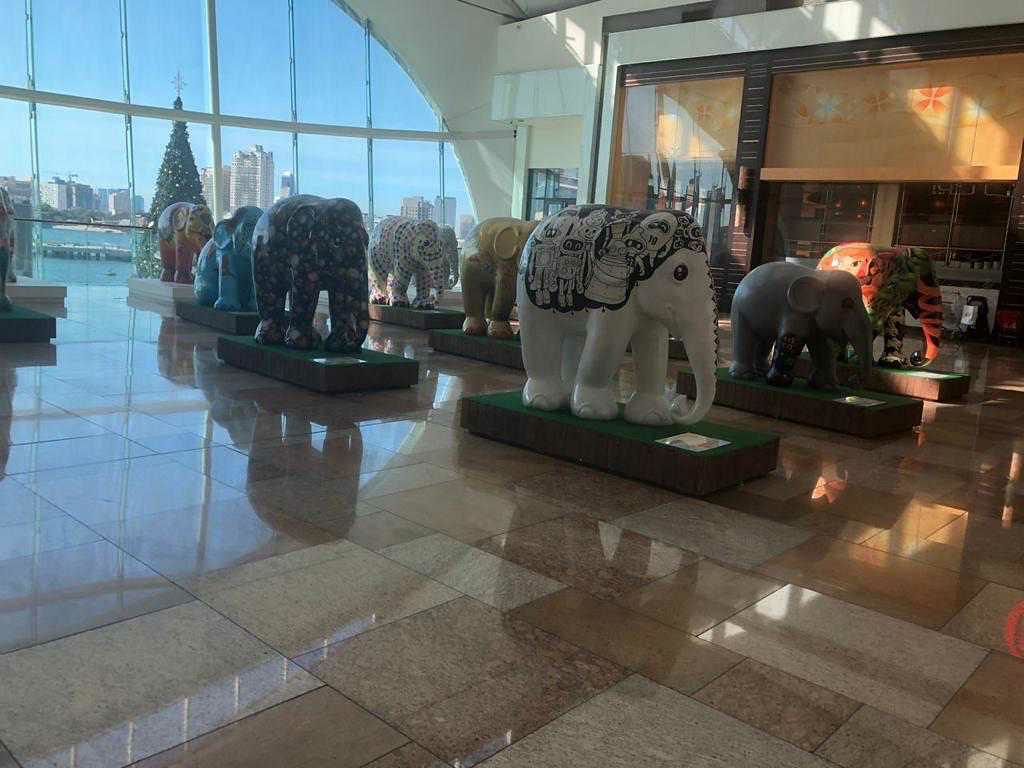This photograph, likely taken inside a metropolitan museum or exhibit space, showcases an array of intricately decorated elephant statues. The statues, resembling baby elephants, are displayed in neat rows on rectangular bases with green tops. Each statue features a unique color and pattern: a white elephant adorned with robots on a black blanket, an all-black elephant with white patterns, an orange elephant painted with a tiger pattern, and an all-gray elephant. The setting is grand, emphasizing polished, reflective tiles in shades of white, cream, tan, brown, and gray. A large, double-story glass window dominates the room, revealing a scenic city skyline, a body of water, and a beautifully adorned Christmas tree with ornaments and a star topper. The elephants, seemingly made of stone and wearing ornate, embroidered coverings, cast shadows on the shimmering floor, enhancing the overall elegance of the scene.